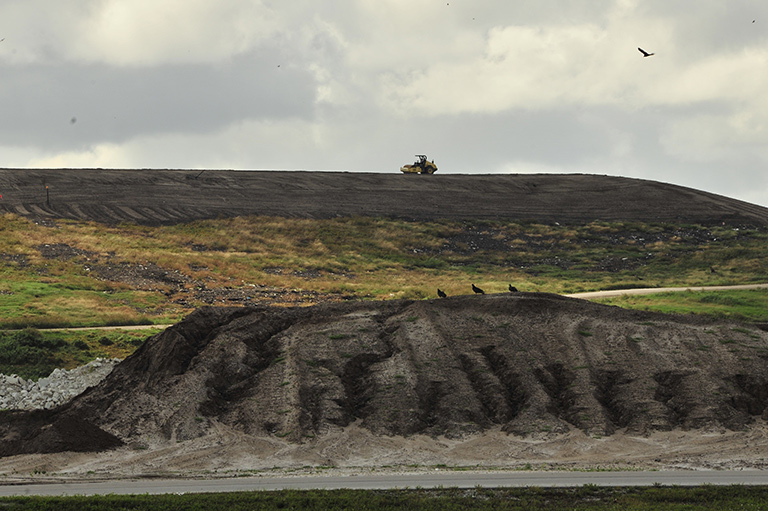The image depicts an overcast day in a quarry or construction area, marked by a series of dirt mounds and gravel piles. In the foreground, a road stretches across the scene, suitable for vehicular travel, flanked by rocky terrain and scrubby, dried grass. Dominating the mid-ground is a substantial mound of earthy debris, atop which three black birds—likely crows—are perched. To the left of this mound, a cluster of rocks is visible. Further back, another road runs parallel to the first, creating a grassy divide scattered with exposed dirt and rocks. Above, on a larger dirt hill, a tractor or steamroller can be seen making its way across the top, suggesting ongoing construction or soil compaction. The sky overhead is densely clouded, casting a gray hue over the entire landscape, and a lone blackbird is captured mid-flight in the upper right of the image.